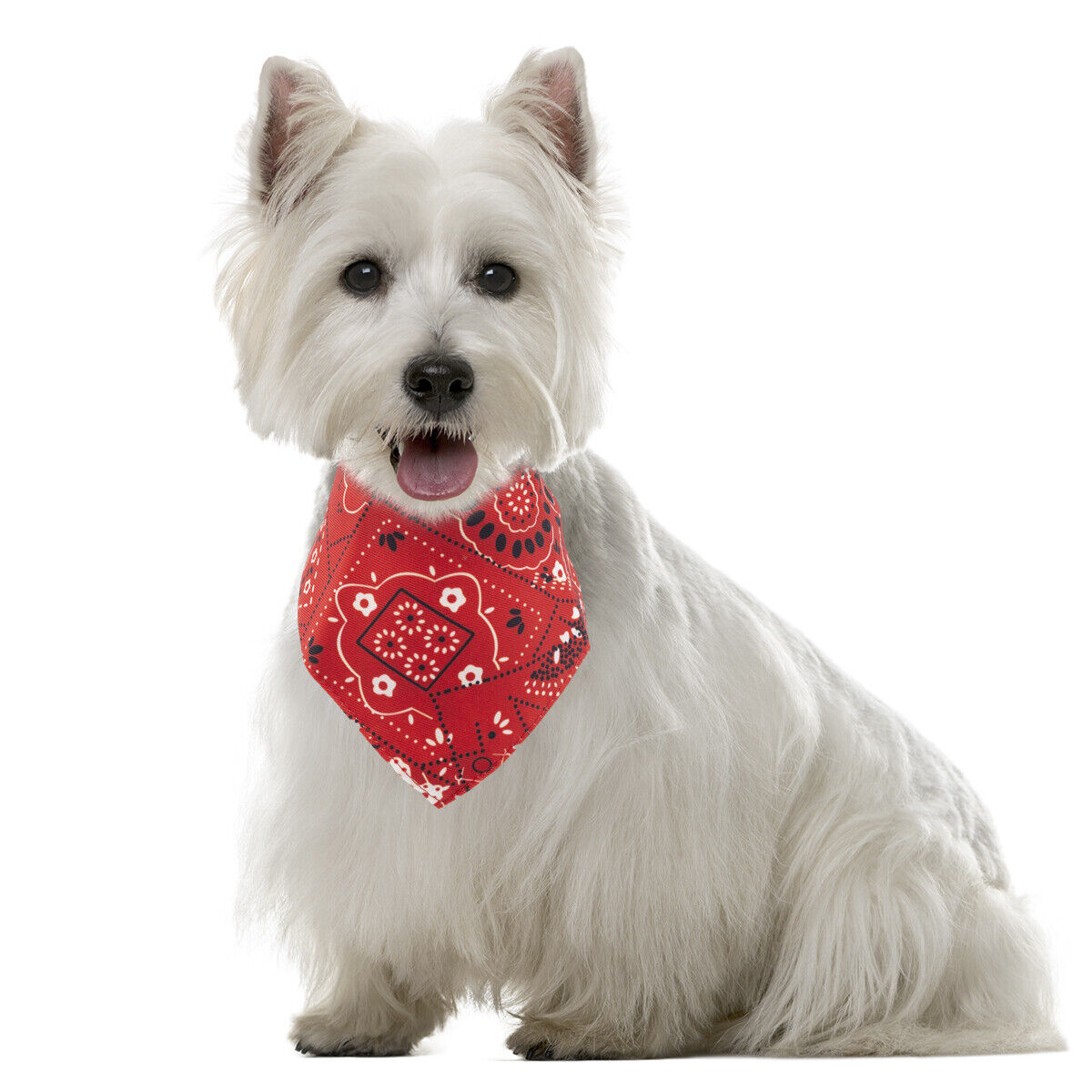This is a detailed picture of a well-groomed, small white dog with long, fluffy fur that drapes over its legs, partially obscuring its little paws. The dog boasts short, pointy ears with extra hair, adding to its adorable appearance. Its tiny, black nose and round, dark eyes radiate a youthful and happy expression. The dog is facing the camera, sitting down with its ears perked up, and appears to be smiling with its tongue sticking out, suggesting a playful demeanor. Around its neck is a red bandana with a classic paisley pattern, although it seems slightly mismatched in size, hinting at possible digital editing. The background of the image is transparent, focusing all attention on the charming, fluffy canine.